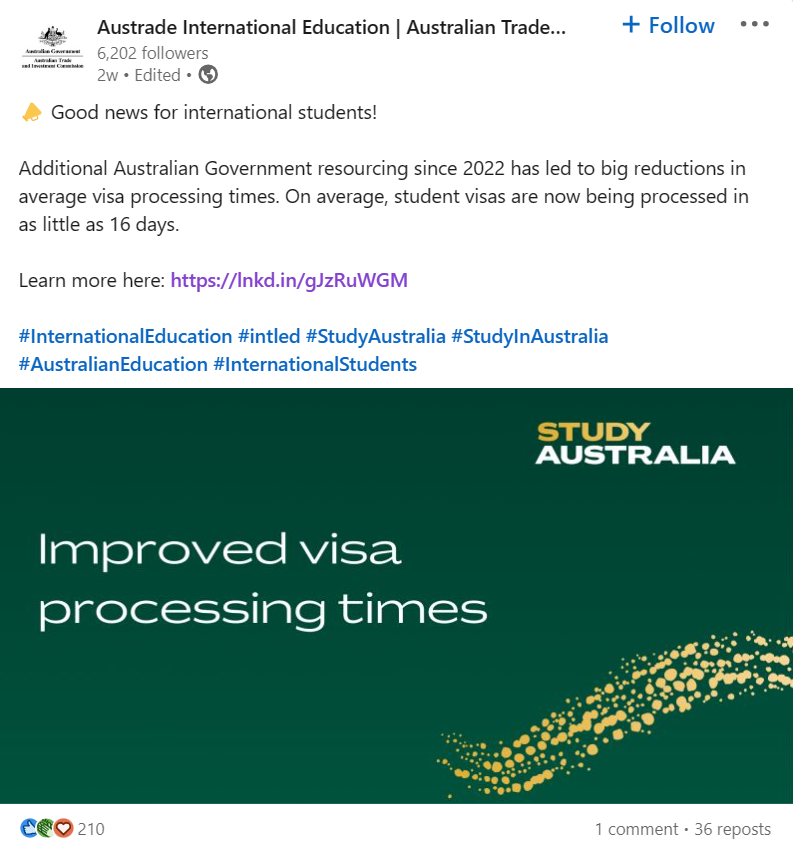This is a detailed description of a screenshot from an unknown source, specifically featuring a post by Austrade International Education on LinkedIn. 

**Caption:**

A screenshot from a LinkedIn post by *Austrade International Education* is displayed. The post highlights significant improvements in the processing times for Australian student visas due to additional government resourcing since 2022. The organization's profile shows 6,202 followers and the content was edited two weeks ago. 

**Main Content:**
The highlighted text exclaims, "Good news for international students!" and explains that the Australian government’s increased resources have significantly reduced the average student visa processing times, now taking as little as 16 days on average. There's a link provided for further information: [https://lnkd.in/gjzruwgm](https://lnkd.in/gjzruwgm).

**Hashtags:**
The post is tagged with several hashtags to enhance visibility: #internationaleducation, #intled, #studyaustralia, #studyinaustralia, #australianeducation, and #internationalstudents. 

**Visual Elements:**
At the bottom of the post, there is a dark green rectangle featuring text that reads, "Improved Visa Processing Times, StudyAustralia." A decorative swirl of golden dots embellishes the bottom right corner of this rectangle.

**Engagement Metrics:**
To the bottom left of the image, engagement icons include a thumbs up, a clapping hands emoji, and a heart, collectively showing 210 interactions. The bottom right corner notes that there is one comment and 36 reposts. 

**Note:**
The screenshot includes no images of people, animals, birds, plants, flowers, or trees.